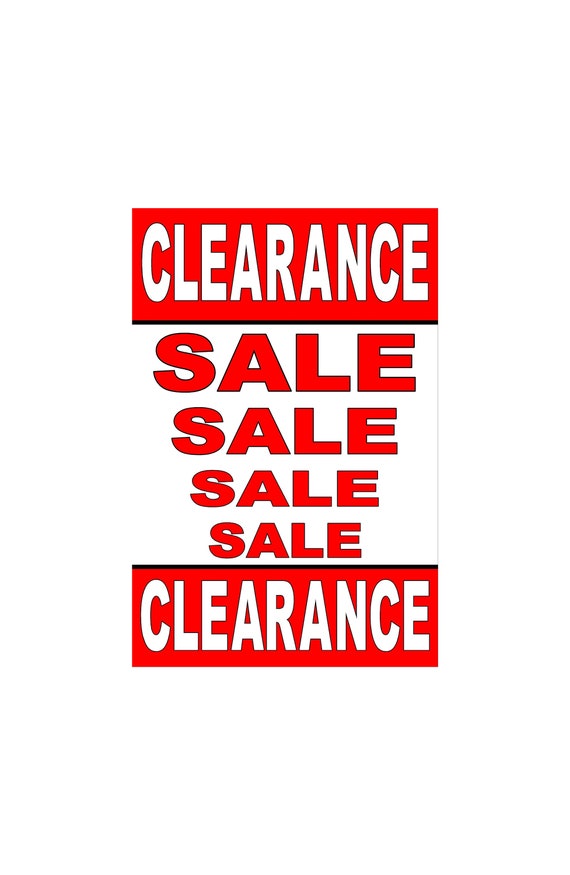This is a vertically oriented rectangular poster designed to advertise a clearance sale. The top and bottom sections of the poster each feature the word "CLEARANCE" in bold, white, capital letters set against a red background. These sections take up about one-fourth of the poster each. Between these "CLEARANCE" sections, there are four occurrences of the word "SALE," displayed in descending order of size, also in capital letters. Unlike the top and bottom sections, these "SALE" words have a red font on a white background. The sales words are arranged to form an inverted pyramid shape, creating a striking visual effect that draws attention. This type of poster would likely be found throughout a store to prominently advertise ongoing discounts.